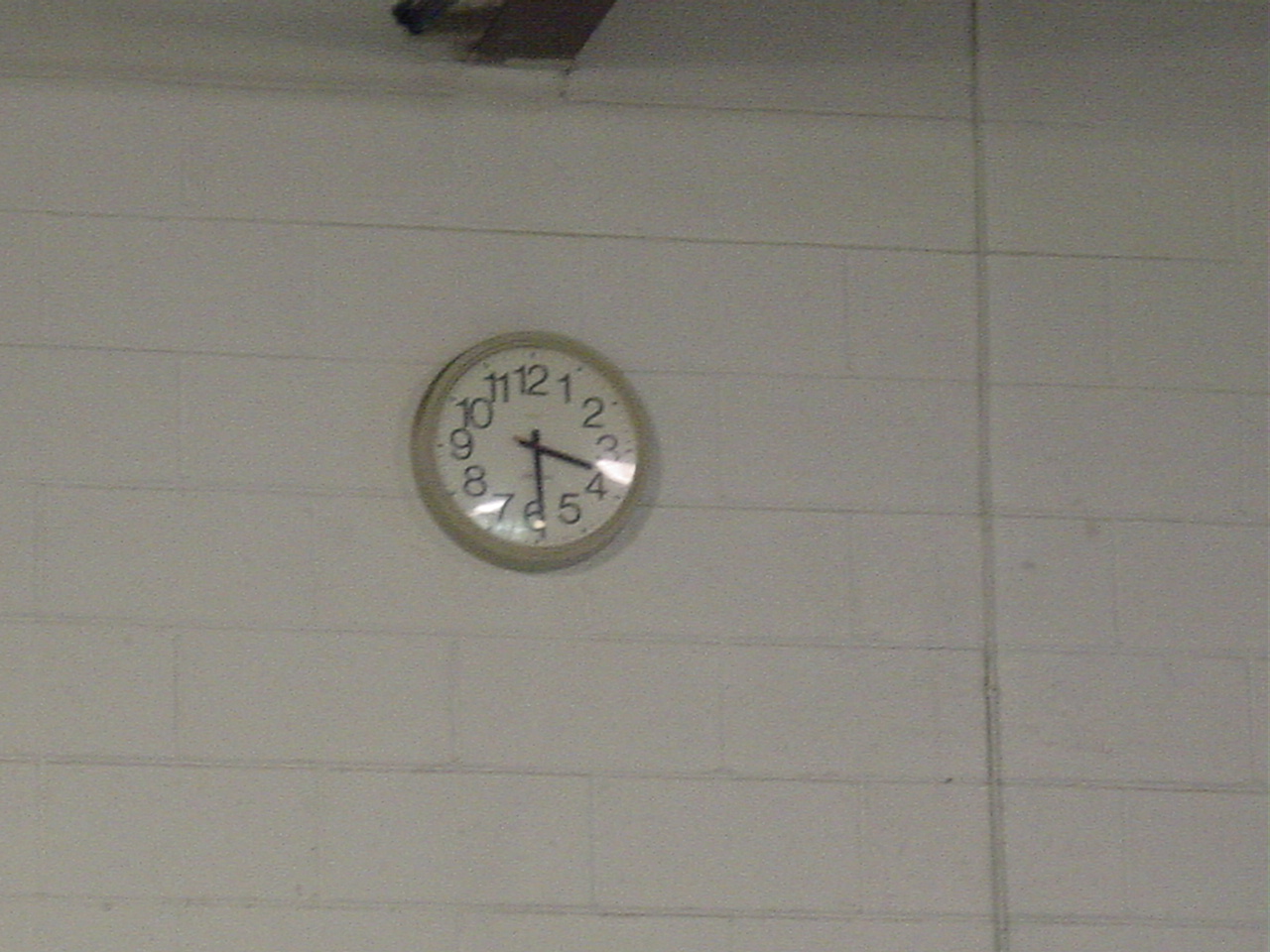A detailed and descriptive caption could be:

"A white wall with a painted brick texture serves as the backdrop for a classic wall clock, which is centrally positioned. The clock, featuring black numerals and black minute and hour hands, is currently stopped at 3:29. Its outer rim, slightly darker and aged, hints at its antiquity. To the right of the clock, a wire descends vertically from the ceiling to the floor. Above the clock, a discolored beam with brown and black stains adds a rugged contrast to the otherwise clean, white wall."